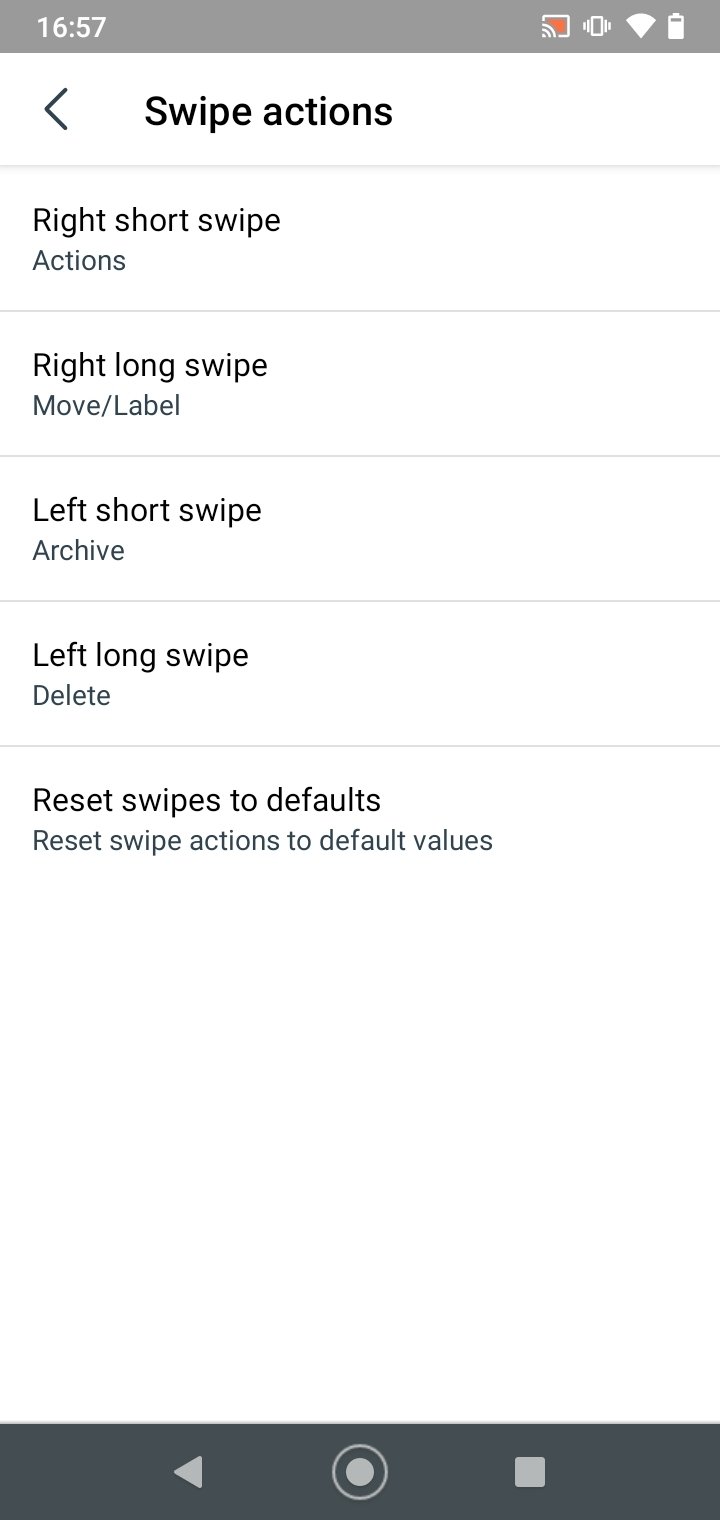The image features a detailed user interface layout. At the top, there is a prominent gray rectangle with the number "1657" displayed on the right side. On the left side of this gray rectangle, there is a white-outlined square containing an orange square inside it. Adjacent to this is a Wi-Fi symbol, and below this, a white-outlined rectangle with smaller lines situated to its side. Additionally, a downward-pointing triangle, rounded at the top, is visible, alongside a battery icon that is mostly full.

Directly beneath this section, the background is white with an arrow pointing to the left accompanied by the text "swipe actions." This is followed by a thin gray line, after which it says "right short swipe actions." Another thin gray line appears and then it says "right long swipe, move - label" followed by another gray line. The text continues with "left short swipe, archive" followed by yet another gray line, and then "left long swipe, delete," followed by one more gray line. Finally, it reads "reset swipes to default," and "reset swipe action to default values."

Towards the bottom of the image, there is a large white space, beneath which lies another gray rectangle. This rectangle features a left-pointing triangle, along with a gray-outlined circle with a light gray inner circle and a light gray square.